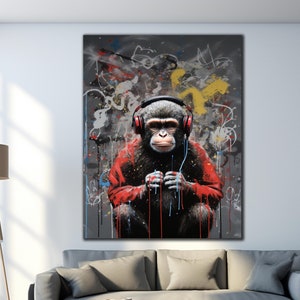This image depicts a modern, minimalist living room with a distinctive piece of art prominently displayed above a gray couch. The painting features a chimpanzee wearing a red jacket and black pants, crouching with its arms resting on its knees and adorned with black headphones with red ear-pieces. The chimpanzee, whose hands are clenched at the knuckles, appears deeply engrossed in music. The background of the canvas resembles a cityscape layered with vibrant graffiti in shades of red, white, yellow, and blue. Notably, the chimpanzee has paint on its hands, suggesting it might have contributed to the mural. The clean, white wall and ceiling of the room, combined with soft natural light streaming from the left side, enhance the clarity of the image and add to the serene ambiance. The couch beneath the artwork is equipped with four throw pillows of varying sizes and colors, further accentuating the coziness of the space.